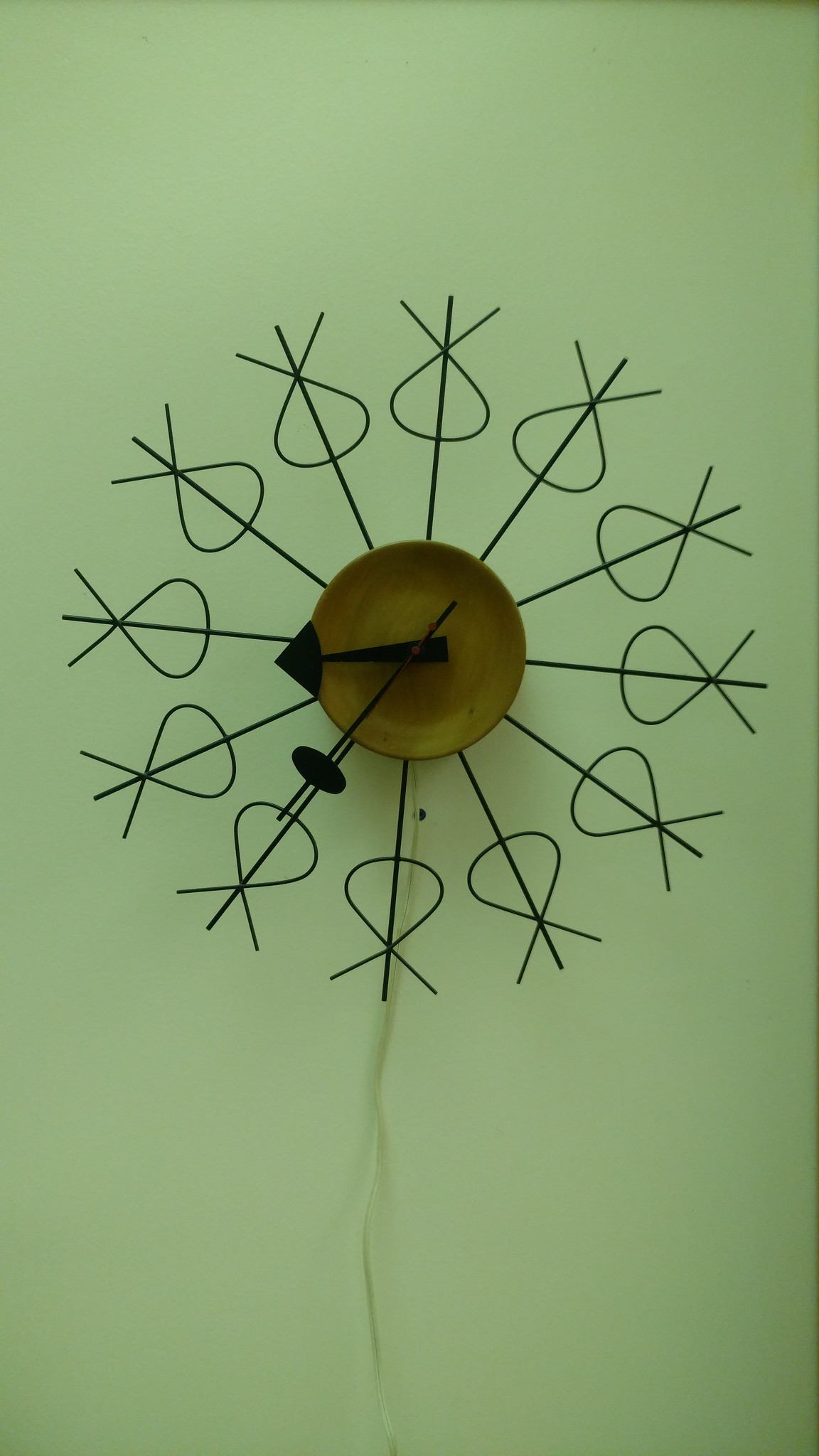The image showcases a modern and minimalist clock mounted on a light green wall. This unique timepiece lacks traditional features such as numbers and a round frame. Instead, it comprises sleek metal rods radiating from the center to form a circular shape. At the end of each rod is a distinctive droplet-like design with two small antennae, which creatively represent the clock's hour markers. The clock is equipped with three hands: one for the seconds, one for the minutes, and one for the hours. The time displayed is approximately 8:36.